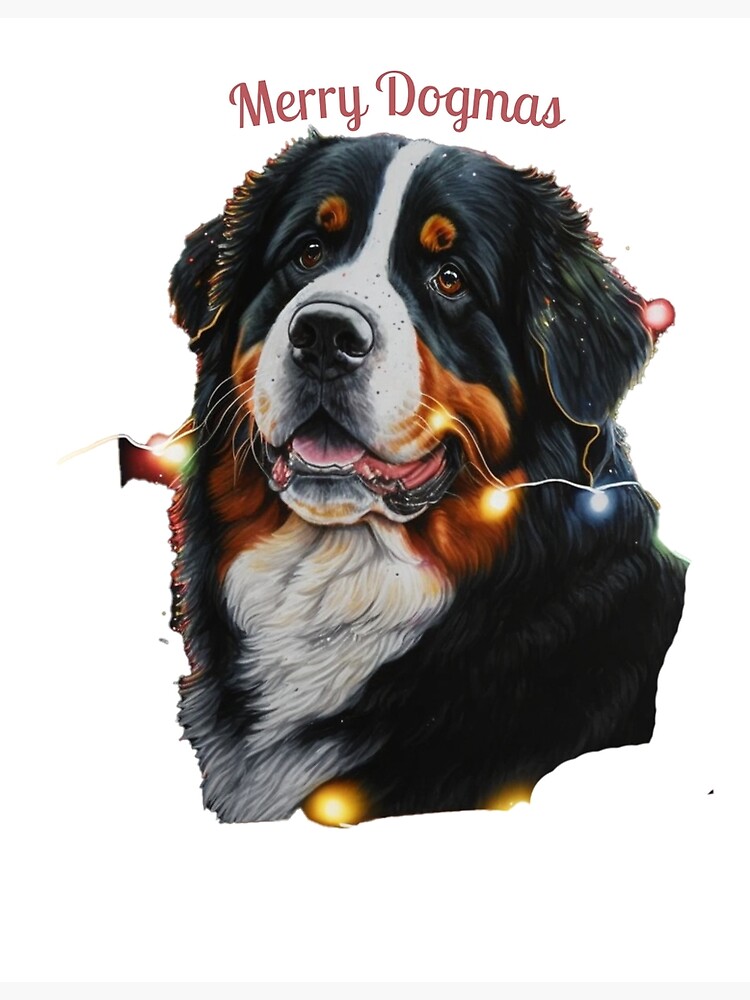This detailed painting features a large, mostly black dog with distinctive white and brown markings. The dog has a white stripe running down the center of its forehead, a white muzzle, chin, and chest. It also boasts brown accents around its muzzle, neck, and chest, with two prominent brown dots above its deep brown eyes. The black-faced canine has a black nose and floppy ears, and appears to be smiling, exuding a happy demeanor. Wrapped around the dog are multicolored Christmas lights in hues of red, yellow, and blue, glowing festively. Above the joyful scene is the playful greeting "Merry Dogmas" written in brownish-red, cursive lettering, framed by thin gray lines at the top and bottom of the image.